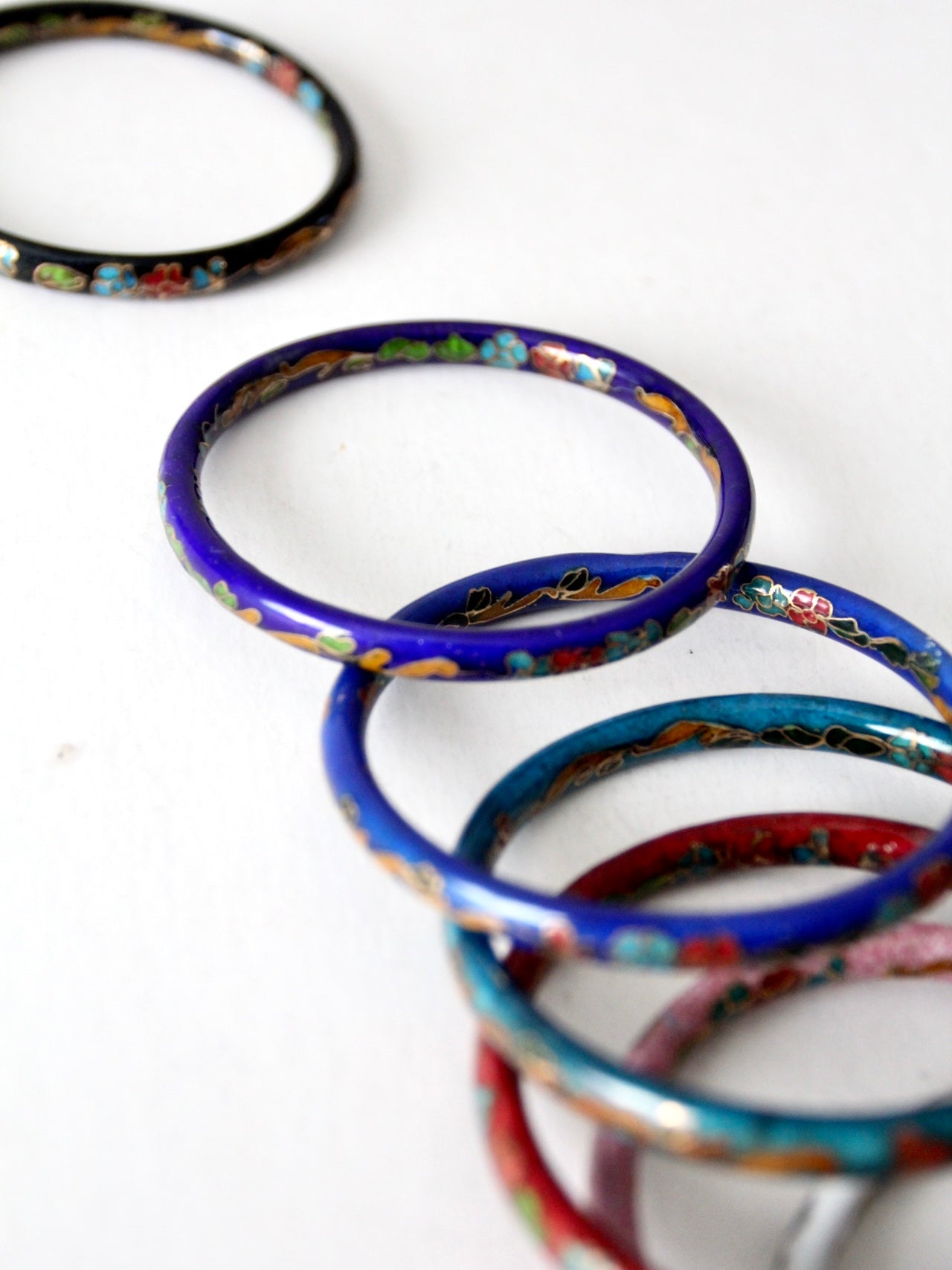This is a detailed photograph of six hand-painted enamel bangle bracelets, arranged on a white background surface. The bracelets feature intricate, colorful floral patterns with gold outlines, showcasing hues of green, yellow, blue, red, and purple. A black bangle, distinct in its position, is situated towards the top left corner of the image. The remaining five bracelets—colored in royal purple, turquoise blue, dark red, peony pink, and another shade of blue—are stacked and intertwined towards the bottom right corner, forming a diagonal composition across the photograph. Additionally, a sliver of a silver bracelet peeks into the frame. The overall arrangement and detailed craftsmanship of the bracelets give off a sense of cultural or artisanal significance, potentially hinting at influences from Native American, Indian, or Moroccan design traditions.